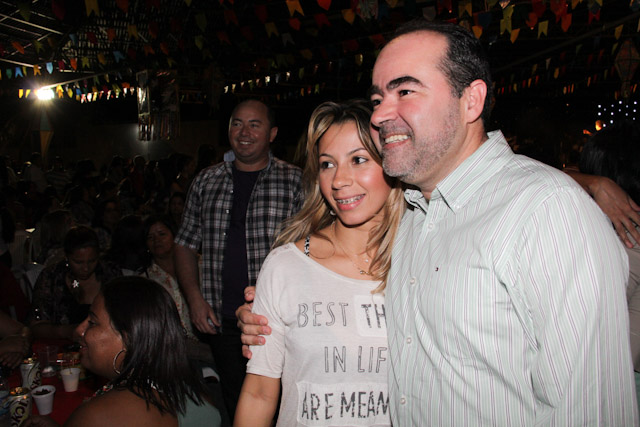In this photograph, a man and a young woman, likely a father and daughter, are standing and smiling inside a bustling, dimly-lit bar or restaurant. The man, with short black hair, bushy eyebrows, and a scruffy beard, is wearing a light-colored, striped collared shirt, and has one arm affectionately placed around the woman's shoulder. She has shoulder-length dirty blonde hair, braces, and is wearing a white t-shirt printed with partially visible text that includes “BEST” and “IN LIFE.” The woman’s cheeks are rosy and she is beaming brightly. They appear to be posing for the camera, looking towards the left of the image. In the background, the room is packed with people, some seated at tables and others standing, indicating a lively atmosphere. Another man, dressed in a flannel shirt over a t-shirt, is also visible smiling behind the main subjects. Scattered cans of beer on the tables, as well as flags hanging from the ceiling, further highlight the festive environment of the scene.